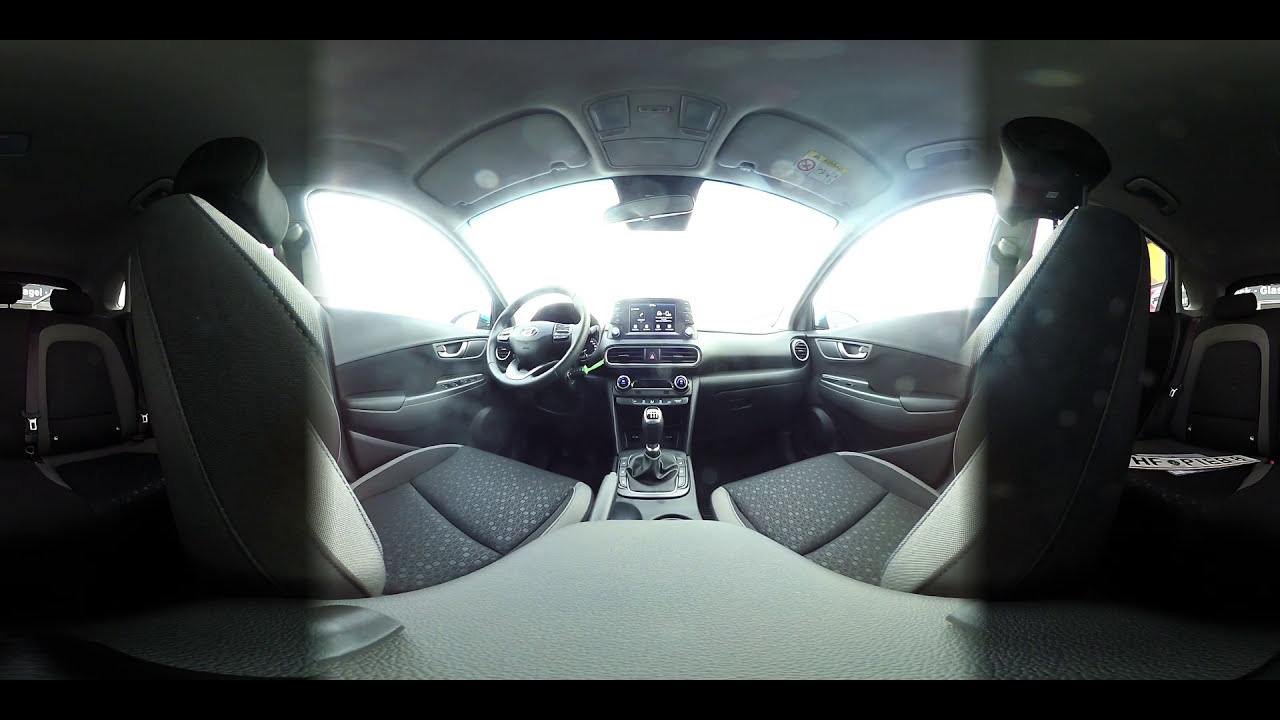This panoramic interior view of a car, specifically taken from the backseat, showcases the detailed layout from the middle section towards the front seats. The sunlight is incredibly bright, flooding through the windows and obscuring any details of the outside world. The vehicle features black upholstered seats with tan trim, a black and gray color scheme throughout the interior, and a silver steering wheel on the left, indicating it's a left-hand driven car. The front seats, visibly unoccupied, are flanked by the driver’s side and passenger side windows, both bathed in sunlight. Notably, the driver’s seat has a black interior with tan trim, along with the prominently black steering wheel. The center console, clearly in view, includes the rearview mirror, the gear shifter, radio knobs, the dashboard, music system, AC vents, and AC controls. Additionally, on the right seat, a number plate with the inscription HF0P1888 can be seen, adding a unique element to the image. The roof of the car is gray, and the bright center contrast sharply with the dimmer edges of this panoramic shot.